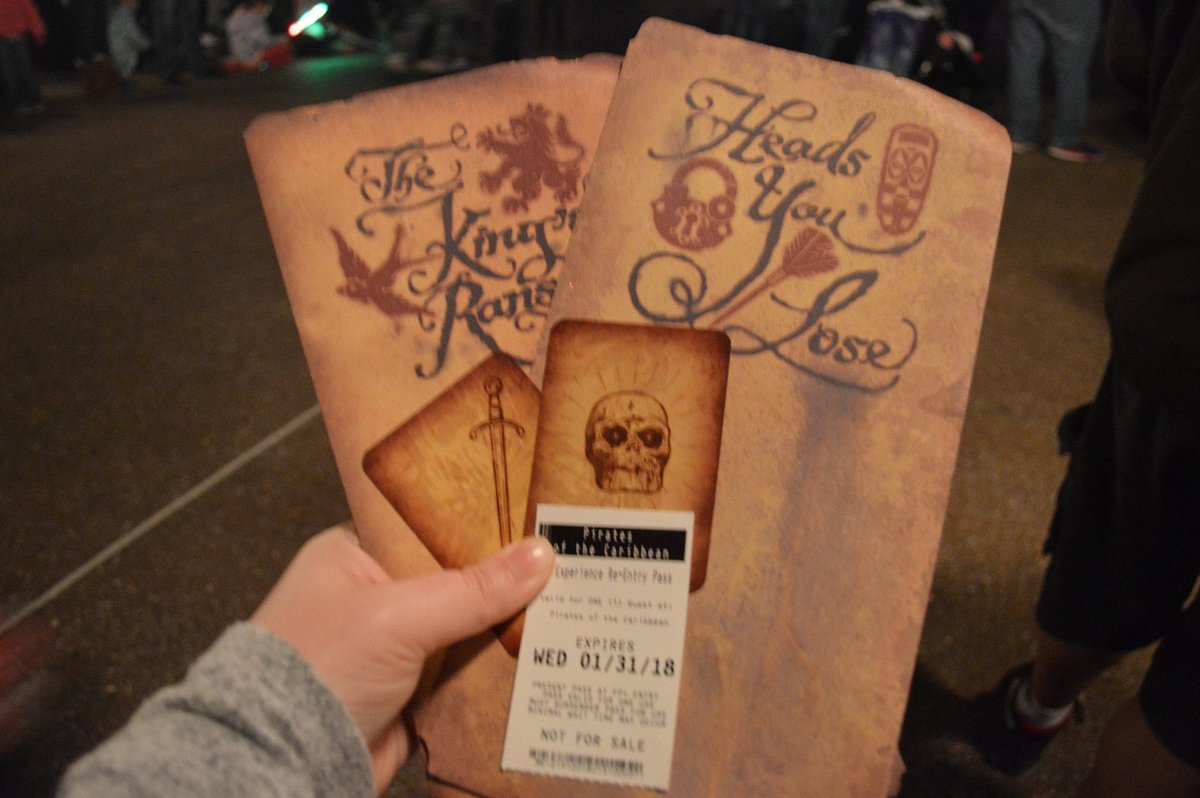In this realistic, horizontally oriented photograph, the focus is on a white left hand emerging from the bottom left corner, dressed in a grey sleeve. The hand holds two ornate, vintage-looking pieces of parchment, approximately 12 to 14 inches tall and 6 to 8 inches wide. The parchment on the left reads "The King's Ransom" and the one on the right says "Heads You Lose," both adorned with calligraphy-style writing. Obscuring parts of the parchments are two playing cards with dark brown edges and light brown centers; the left card features a sword illustration, while the right displays a skull. Atop these cards, held under the person's thumb, is a white ticket or receipt with black text, prominently stating, "Expires Wed 01-31-18." In the blurred background, there is pavement and indistinct figures, possibly indicating the photo was taken at an event, where someone nearby appears to be holding a green glow stick.